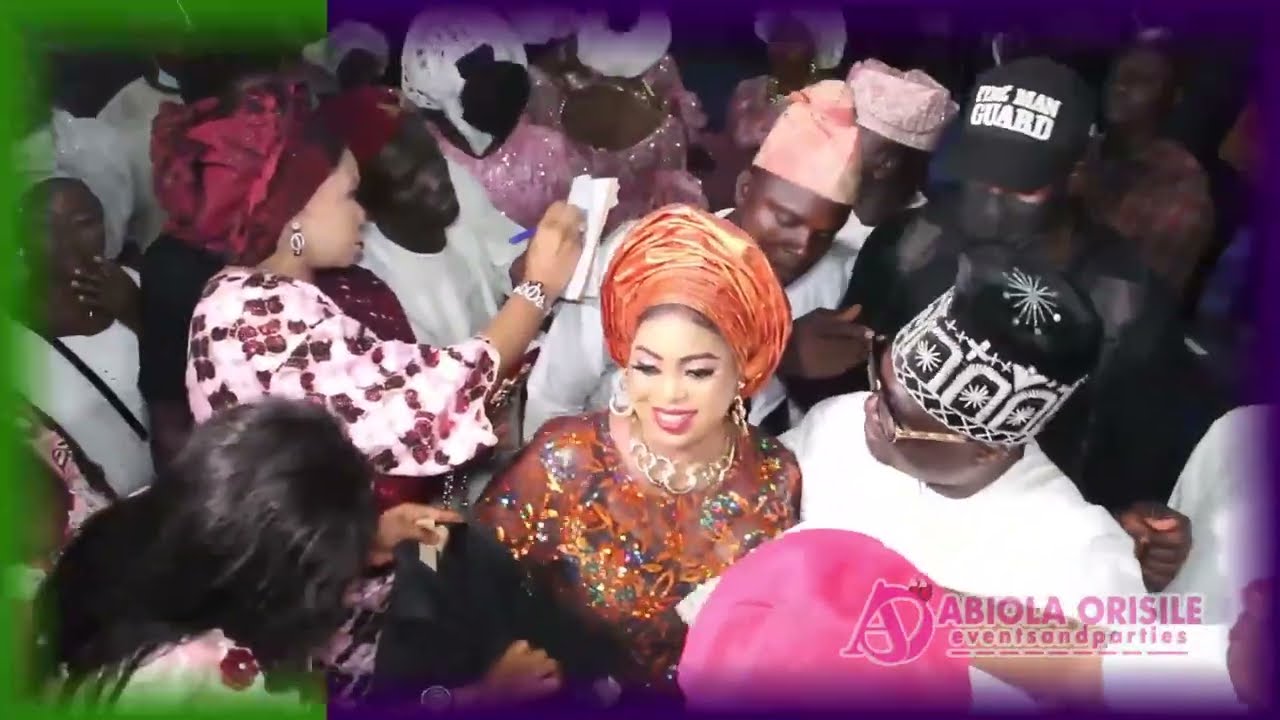The image depicts a crowded scene viewed from above, focusing on a central woman with an elaborate, tall orange headdress resembling a turban. She has brown hair adorned with gold earrings and a shiny gold necklace, and she's dressed in a multicolored, ornate blouse with a maroon base and intricate designs. Her bright lipstick and eye mascara accentuate her smile. Surrounding her are numerous individuals, mostly wearing white clothing and various types of headwear, suggesting religious or cultural significance. Notably, a man in a black hat with white lettering that reads "MAN GUARD" stands out. Another woman to the upper left is elegantly dressed in white and maroon with a tall hair covering, seemingly signing an autograph. The scene is bustling with people facing in multiple directions. At the bottom right, a watermark reads "ABIOLA ORISILE EVENTS AND PARTIES." Amidst the crowd, there are elements like a single arm reaching in from the lower right corner and a partial view of a person with black hair in a floral white garment at the lower left. A green haze or coloring borders the left and top edges of the image.